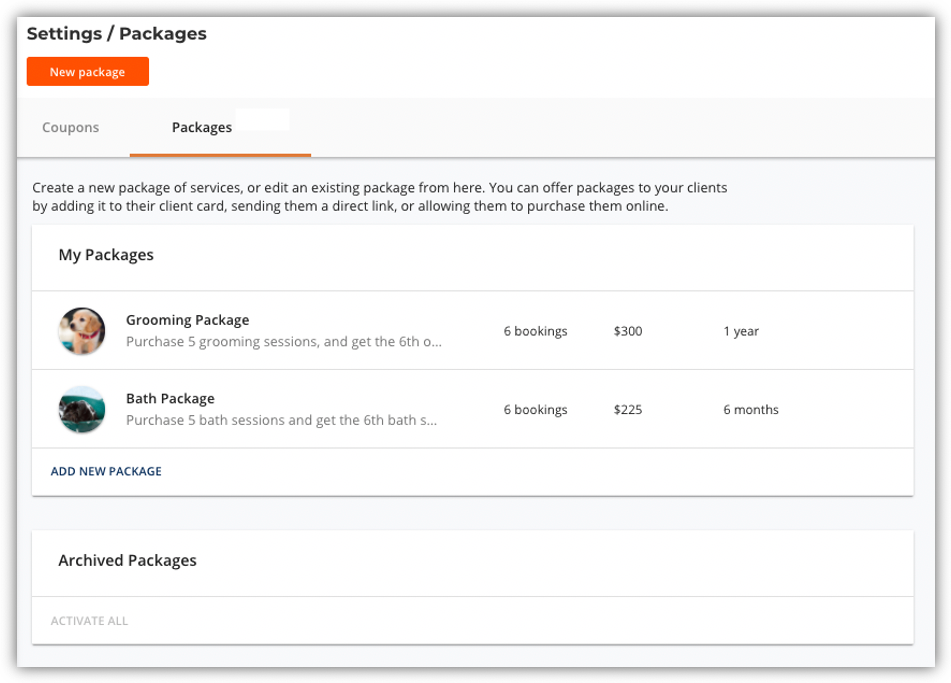Screenshot of a Website Featuring Package Management Options

The screenshot showcases a website's package management section against a light blue background. At the top, the section heading reads "Settings / Packages" with "Packages" underlined in orange. To the right, there's an orange rectangle button labeled "New Package" in white text. Below the heading, a description explains that users can create new service packages or edit existing ones. It also mentions that these packages can be offered to clients through various means: adding them to a client card, sending a direct link, or allowing online purchases.

The section is organized into different package options. The first is labeled "My Packages" which includes various service packages such as:

1. **Grooming Package**
   - **Image:** A picture of a dog.
   - **Description:** "Purchase five grooming sessions and get the sixth one free."
   - **Details:** "O... 6 bookings, $300 for one year."

2. **Bath Package**
   - **Image:** An ocean scene.
   - **Description:** "Purchase five bath sessions and get the sixth session free."
   - **Details:** "S... 6 bookings, $225 for six months."

Additional options at the bottom of the screen include buttons for "Add New Package," "Archive Packages," and "Activate All."

The interface is designed to guide users through the process of managing and offering service packages to clients efficiently.